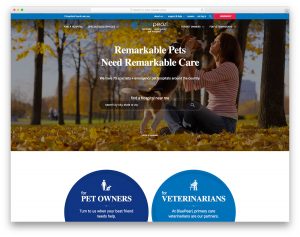This screenshot is of an image that captures a serene and bucolic scene, albeit difficult to read due to its small size. Central to the image is a woman seated on a leafy forest floor, adorned in a striped red shirt and blue jeans. She sits cross-legged, oriented towards the left of the frame, but positioned more towards the right side. The woman is gently lifting a beagle puppy by its front legs, its back paws still touching the ground, while she makes a kissy face at the adorable canine. Surrounding them are rows of tall trees, whose branches begin several feet above the ground, adding to the peaceful ambience of the scene. Complementing this picturesque moment, overlaying white text at the top reads, "Remarkable pets need remarkable care." At the bottom, a white section features two blue circles: a dark blue circle on the left inscribed with "pet owners" in white text, and a lighter blue circle on the right that says "for veterinarians."